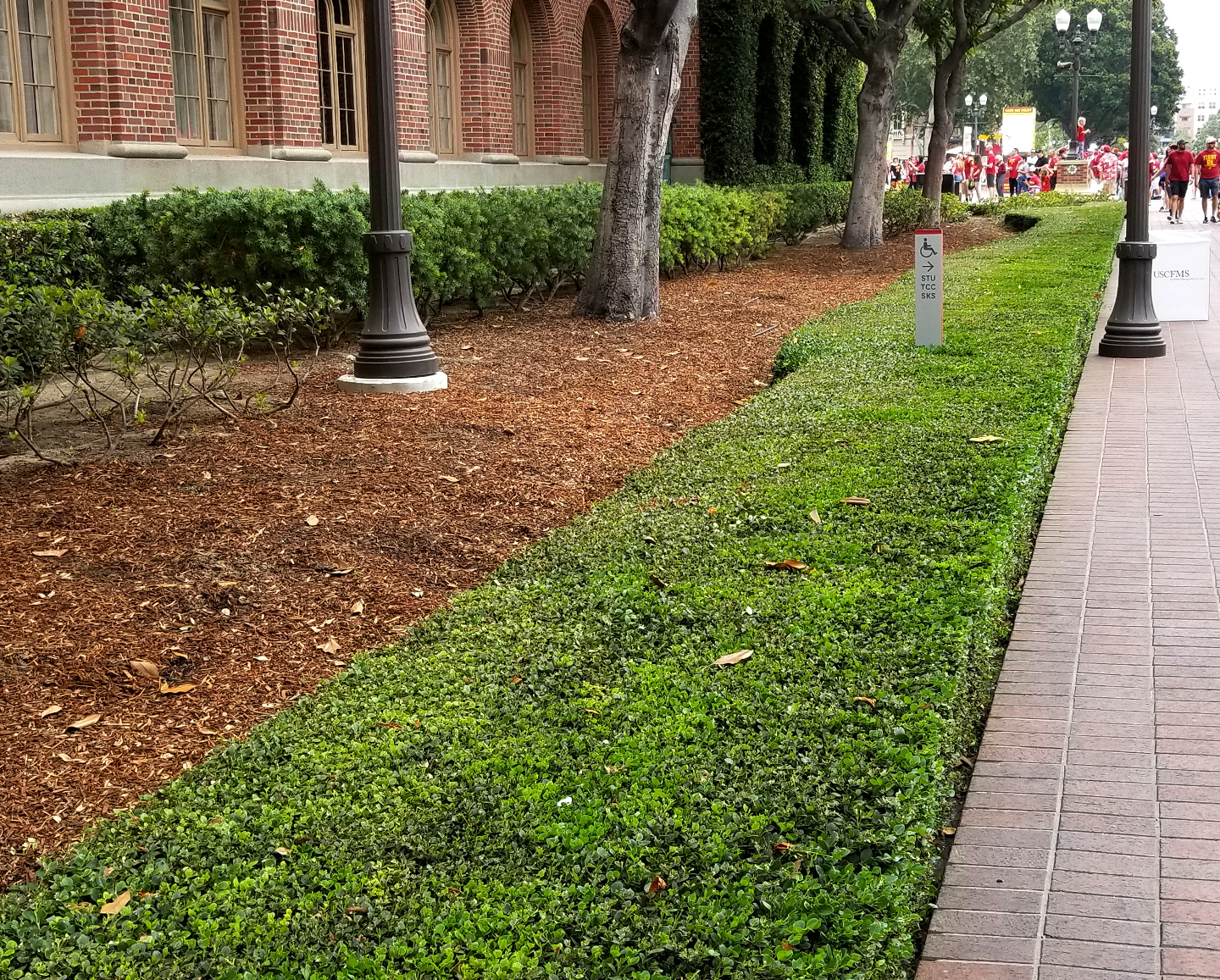The image captures the exterior of a red brick and cement university building, partially visible in the background. A meticulously maintained landscape adorns the scene with neatly trimmed hedges running diagonally from the bottom left to the top right. In front of the building, a combination of green grass and mulch beds, filled with various foliage, adds to the well-groomed aesthetic. Interspersed within the mulch are street lamps and a handicap sign featuring a wheelchair symbol. The brick walkway, lined with closely edged grass, guides a flow of pedestrians, many dressed in red, possibly coming from a sporting event. A row of green bushes continues behind a tree trunk and lamppost, with pillars extending across the building's façade, completing the structured and orderly environment.